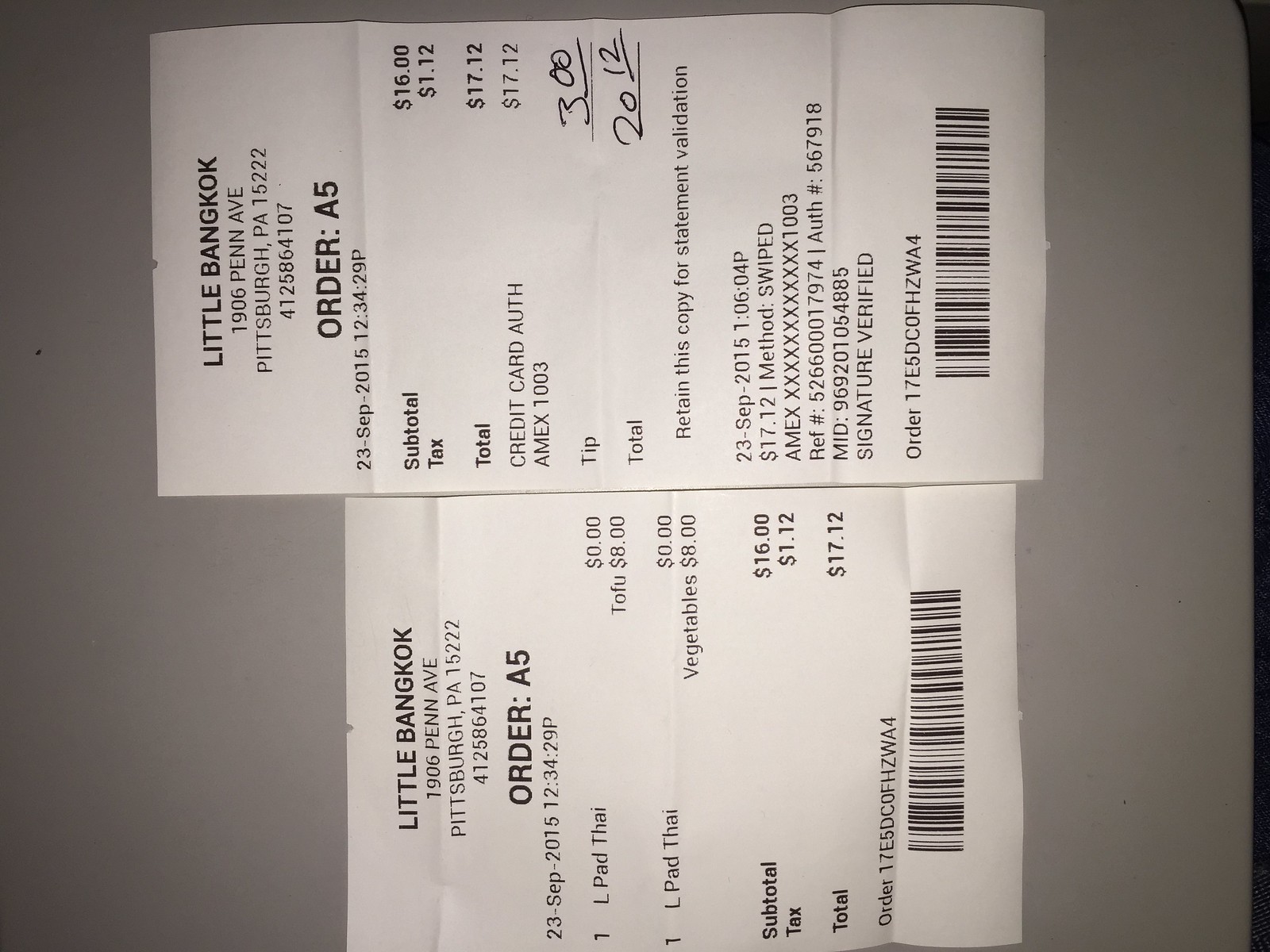"This photo features two receipts from Little Bangkok, a restaurant located at 1906 Penn Avenue in Pittsburgh, Pennsylvania. The receipts are oriented sideways with their top edges facing left. The first receipt, labeled 'Order A5,' is longer than the second and lists two items: 'L-Pad Thai' with tofu priced at $8 and 'L-Pad Thai' with vegetables also priced at $8, summing up to a total of $17.12. The second receipt, a copy of the first, includes an additional $3 tip, bringing the total to $20.12. Payment was made using an American Express credit card."